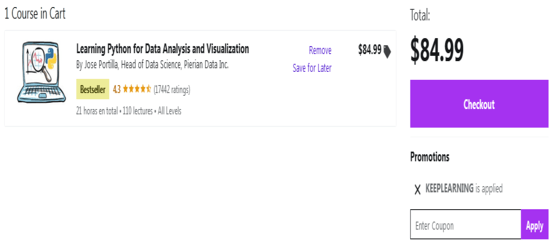The image captures a screenshot of the cart section from an online education platform. The background is predominantly white, emphasizing a clean and simple layout. At the top left corner, it indicates "1 course in cart." Below this, there is a thin, gray border outlining the course details.

The course featured is "Learning Python for Data Analysis and Visualization" by Jose Portilla, Head of Data Science at Data Inc. This course is marked as a bestseller with an overall rating of 4.3 out of 5 stars, based on 17,442 ratings. A cartoonish drawing of a light gray laptop, displaying a magnifying glass on its screen, visually represents the course. 

The course includes 21 hours of content across 110 lectures, suitable for all levels. To the right of these details, there are two purple buttons labelled "Remove" and "Save for later." The course is priced at $84.99, with the total cost reiterated at the top of the cart section.

Below the total cost, there is a prominent purple "Checkout" button. Additionally, a promotional message stating "Keep learning is applied" is visible, alongside a coupon input box and an "Apply" button, both located at the bottom right of the screen.